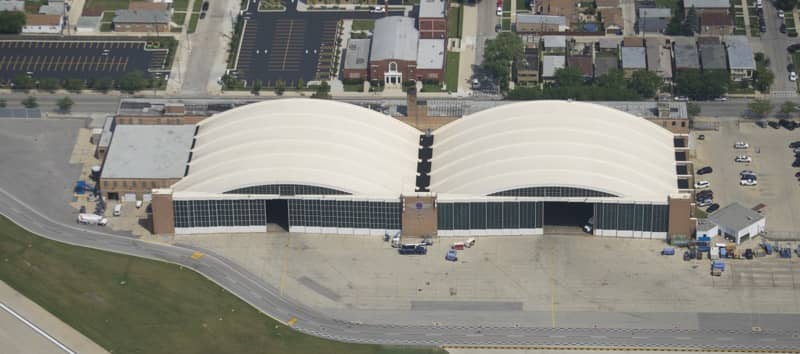The image is a detailed aerial view, likely captured by a drone, featuring two side-by-side aircraft hangars with distinctive white, curved rooftops. The hangar on the right is more open than the one on the left, and both have dark structures between them, contrasting sharply with their white roofs. In the foreground, in front of the hangars, there is a runway marked with white dashed lines. 

To the right of the hangars, there is a parking lot with several cars, adjacent to a small square building. Behind this parking lot, more buildings are visible, including additional smaller structures and residential areas. The top left of the image shows two empty parking lots with yellow lined demarcations on blacktop.

To the left of the hangars, there is a larger square building with a few trucks parked around it, and a winding road that leads downhill, seemingly towards an airfield. In the background, particularly behind the hangars, there are additional buildings, with some residential homes visible on the top right side, lined with trees.

The entire scene spans over two city blocks, blending industrial architecture with surrounding smaller buildings and residential areas, underscoring the vast size and diverse use of the terrain.